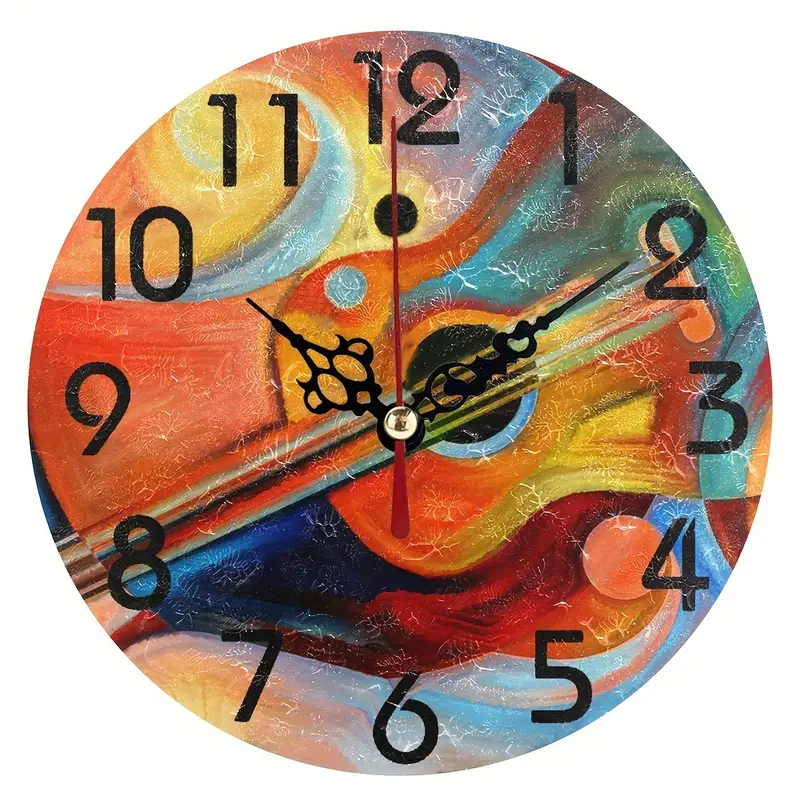This image depicts a round wall clock with a vibrant, watercolor-style background that features a guitar angled across the clock face. The guitar neck is oriented towards the number eight, while the body extends from between the numbers one and three. The clock's background features a swirl of bold, multicolored hues—blues, oranges, reds, and yellows—arranged in a way that resembles a Métis color pattern. The clock hands are ornate and black, with the hour and minute hands resembling intricate keys, and the second hand is a solid red. The numbers on the clock are large, bold, and black in a slightly cursive font, making them easy to read. The clock face reads slightly differently as to the exact time, but it is approximately 10:09 or 10:10. The design includes additional artistic elements, such as blocks of color and a white swirl reminiscent of a moon, all set against a white backdrop.